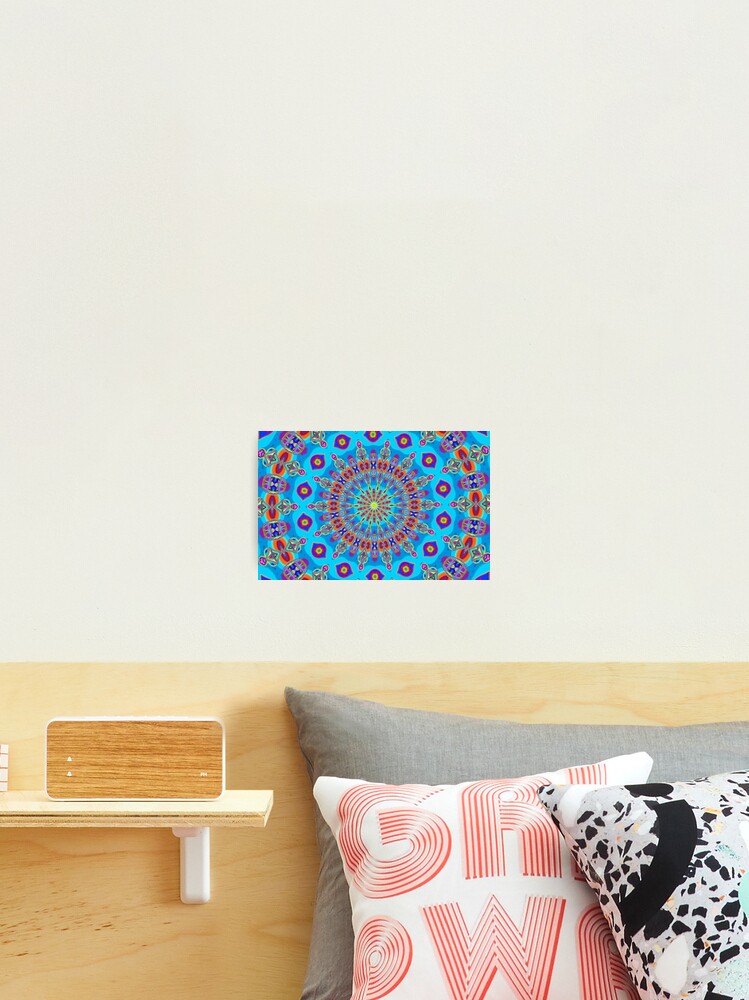The image depicts a cozy indoor setting with a white, possibly off-white, wall as the backdrop. Centrally mounted on the wall is a vibrant, geometric painting reminiscent of a kaleidoscope. This artwork features an array of colors including red, blue, yellow, pink, and orange, with intricate circular designs that resemble spinning purple eyes encircled by yellow dots and extending outward like a carousel. Below the painting is a light wood headboard, indicating the presence of a bed accompanied by several distinct pillows. To the left, there's a gray pillow, while in front of it, a white pillow with red text spelling "G-R-L-P-W-R" adds a pop of color. To the right, another pillow in white with black linings and dots completes the arrangement. Adjacent to the bed on the left side, a small shelf with a wooden radio or box, featuring light colored wooden paneling and white accents, adds to the room's intimate and personalized atmosphere.